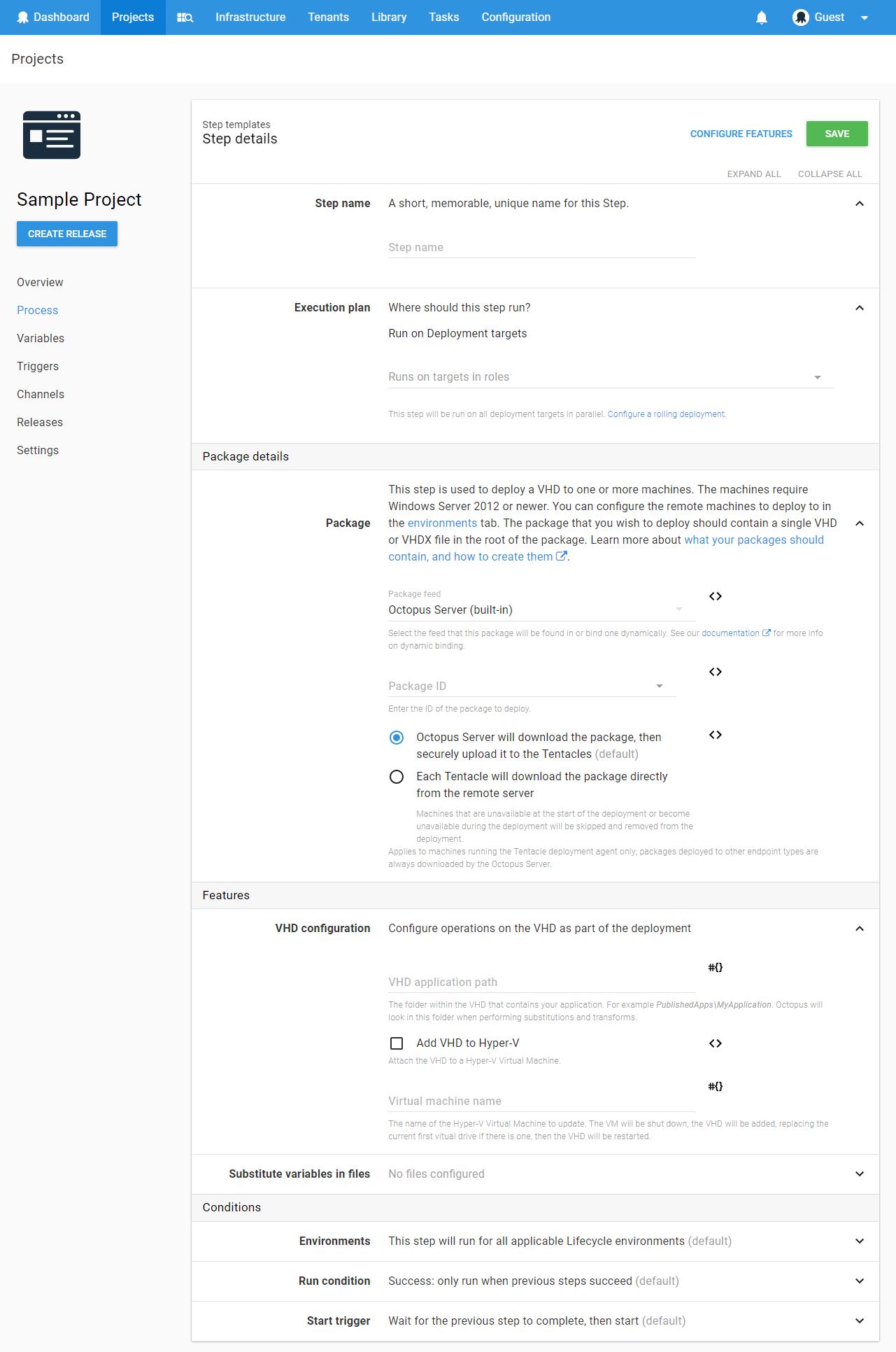The image depicts a section of a website specifically dedicated to project management. At the top of the interface, a blue navigation bar features various tabs, including "Dashboard," "Projects," "Instructions" (although it's unsure if this is exact), "Library," and several other options that are difficult to discern. In the top right corner, there is an indication of a guest profile, complete with a profile picture.

The main section of the page is titled "Step Details," offering detailed instructions on how to perform specific tasks within the project. Prominently highlighted in blue, a section labeled "Features" stands out, and a green "Save" button is visible for preserving changes made.

The central area is organized into several input fields including "Step Name," "Execution Plan," and "Package Details," with some form of inline instructions or placeholders written in black and clickable blue inserts for additional options or links. A service named "Octopus" appears to be a focal point, with one of its steps or cycles highlighted in blue, indicating its importance or current status.

Further down, the page continues to elaborate on "Features" in black text, listing details such as "Substitute Variables in Flex." The section on conditions at the bottom of the page outlines three specific conditions, each clearly enumerated to guide the user through creating or managing their project workflow effectively.